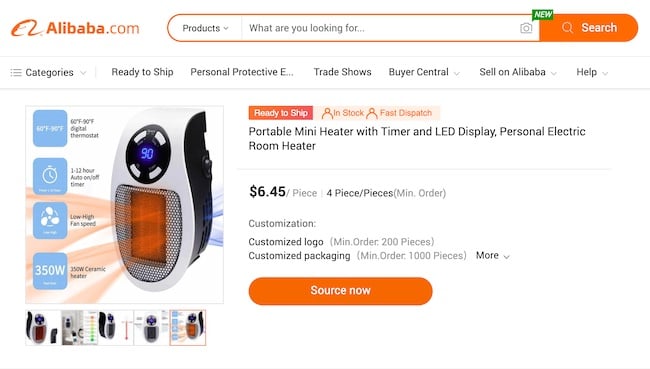This is a cropped screenshot of a product page on the desktop version of the Alibaba.com website, featuring a clean white background. At the top left, the orange Alibaba.com logo is prominently displayed. Adjacent to the logo is an expansive search bar. On the left side of the search bar, a drop-down menu is set to "Products". Within the search bar, the placeholder text "What are you looking for?" is subtly written in small gray font. To the right of the text, there’s a camera icon, indicating a photo search feature, highlighted by a small green box labeled "New". Further to the right, a conspicuous orange search button features a magnifying glass icon on its left.

Beneath the header, a horizontal list of categories spans the top of the page. The categories include "Categories" with a drop-down menu, "Ready to Ship", "Personal Protective Equipment", "Trade Shows", "Buyer Central" (also with a drop-down menu), "Sell on Alibaba" with its own drop-down menu, and "Help", which also contains a drop-down menu.

On the lower left of the screenshot, there is a large thumbnail image of a portable mini heater. The thumbnail displays the heater on the left side, with four blue squares to the right highlighting key features. Below this primary thumbnail, there are five smaller square thumbnails, with the fifth one bordered in red to indicate that it’s the active selection. To the left of the thumbnails, detailed information about the product is listed, including description, price, quantity, customization options, including logo and packaging, and other relevant details. At the bottom of this section, a large orange button labeled "Source Now" prompts users to take action.